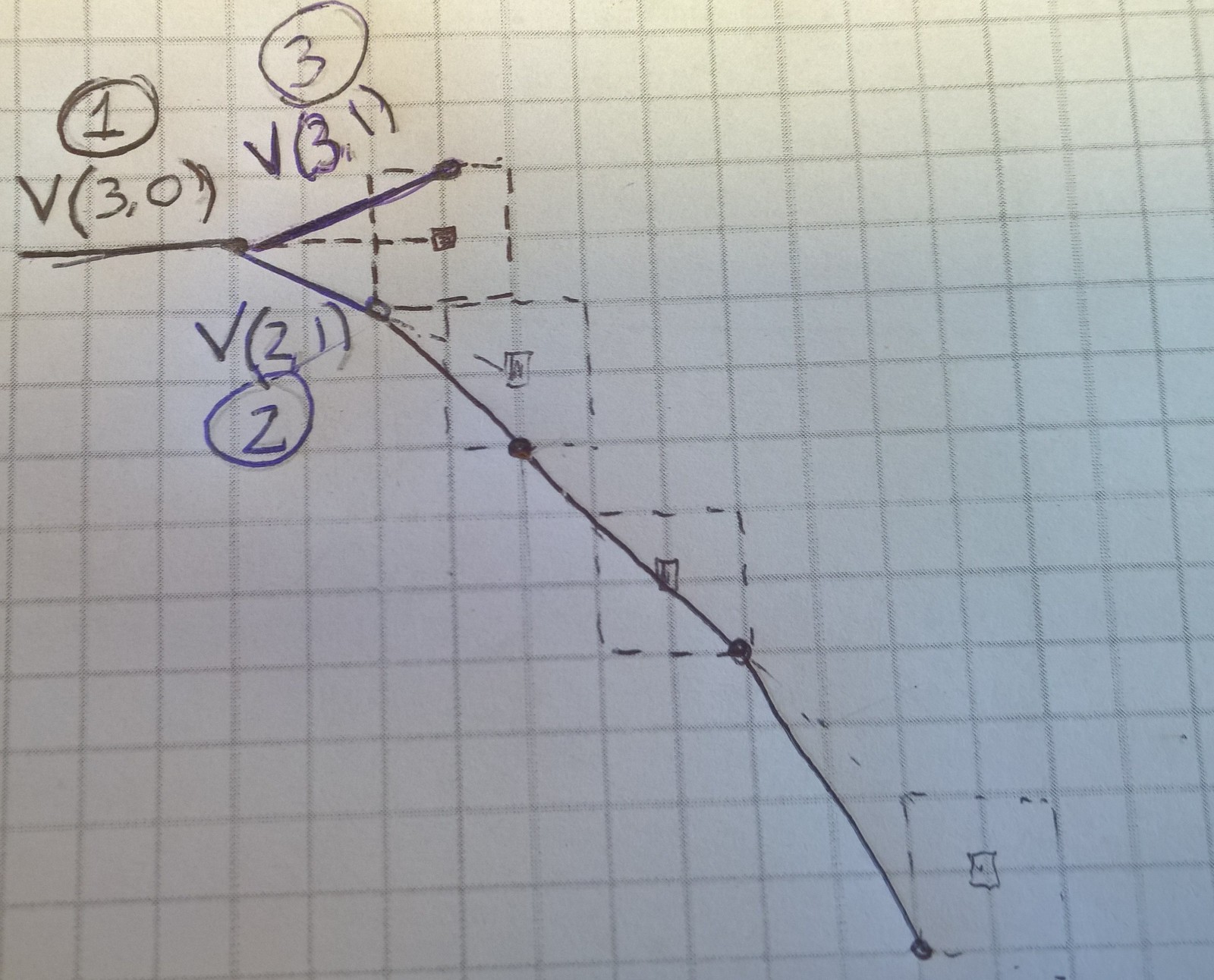This is a detailed close-up illustration of graph paper. The paper is white with gray intersecting lines that form a grid of white boxes. A line starts near the top-left corner, traveling horizontally for three boxes before descending diagonally across multiple boxes, ultimately ending near the bottom-right corner. At the top of the graph paper, the top line is labeled "V(3,0)," with a circled numeral "1" positioned to its right on an adjacent line that extends upward for the space of three boxes. Further down, there is another label, "V(3,1)," with a circled numeral "3" above it. Various colors of ink, including blue, dark purple, and possibly black, were used in the drawing. Dots mark the line's descent to the bottom, culminating in an ending dot. Along the line, there are adjacent or overlapping boxes drawn in dotted lines, totaling at least four boxes. The labels "V(2,1)" and a circled numeral "2" appear below the other "V" points, indicating additional points of interest on the graph paper.